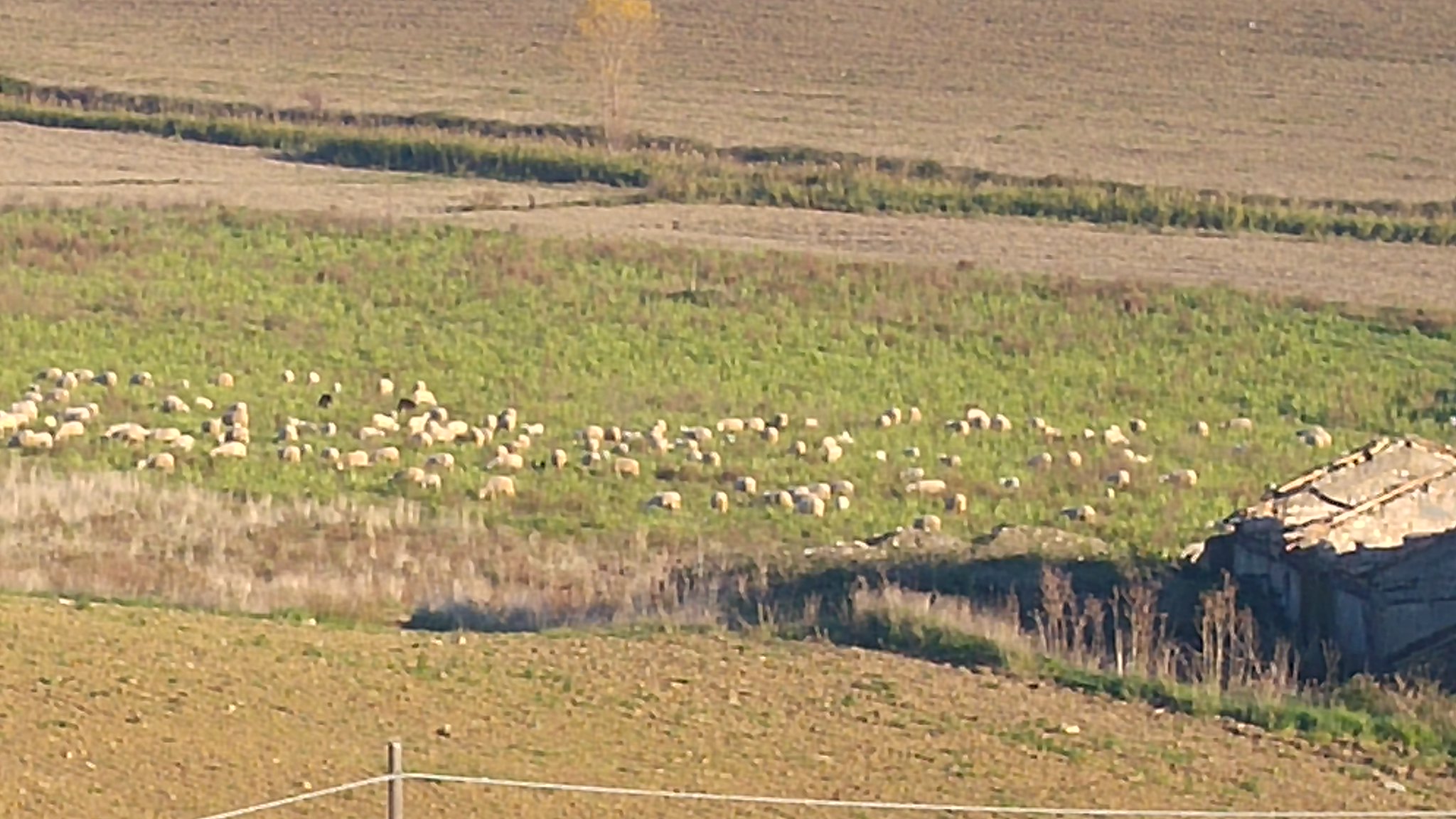The photograph captures a sprawling, low grassy plain extending into the distance. In the foreground, patches of bare brown dirt intermingle with sparse, struggling tufts of grass. To the right, a prominent, shadowed gray rock juts into the scene, surrounded by taller, desiccated grass. Just beyond the rock, a rope fence anchored by a wooden stake adds texture to the landscape. The central band of the image features a verdant strip of green grass teeming with around 50 to 100 white and beige sheep, some lying down, others grazing, their forms scattered from left to right. In the far distance along the top, the landscape transitions to a swath of bare dirt interspersed with grass, punctuated faintly by an ancient, dilapidated shed that appears to be collapsing. Distant yellowish trees subtly frame this bucolic, sun-weathered field, enveloping the scene in a pastoral charm.